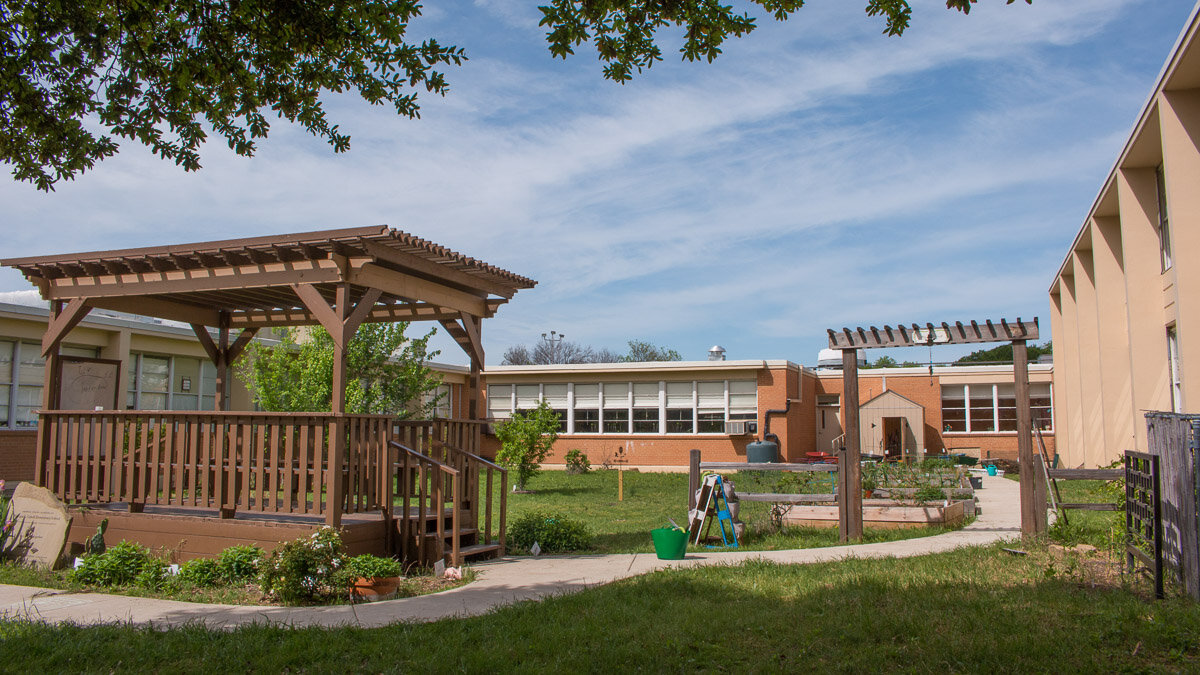The image captures an outdoor scene of a one-story building that resembles a school but could also be a retirement home or office. The background showcases a well-maintained backyard area with a variety of distinctive features. On the left side, there's a brown, oblong-shaped wooden gazebo with railings all around and a set of three steps leading up to it. This gazebo is surrounded by grass, bushes, and a decorative big rock, along with a few plants in the ground and potted plants by the stairs. Directly ahead in the center, there's a green bucket placed on the sidewalk, next to which is a tripod-like structure indicating some ongoing activity. To the right of the bucket, there's a ladder with blue and metal steps. Further right, a wooden archway serves as an entryway, connecting the sidewalk to the building itself. The building features brownish-tan walls, white-framed windows, and an open door leading to a small shed. Overhead, tree leaves hang down and the sky is blue with white clouds, adding to the serene ambiance of the scene.